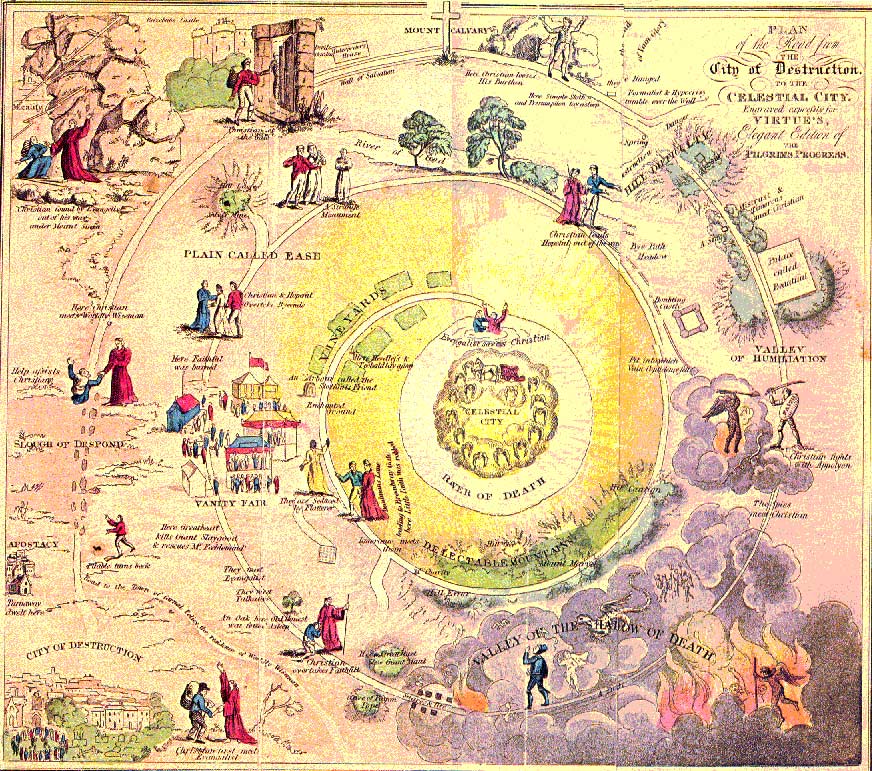This image appears to be an intricate, medieval-style map that vividly illustrates a journey of life with detailed representations of various stages and challenges. The entire composition is square and framed by a light, color-shifting border. At the heart of the image is a golden, orb-like center labeled "Celestial City," surrounded by a corkscrew or swirl design in muted pink and yellow tones symbolizing the "Path of Death." Concentric circles emanate from this center, outlining a spiraled path through life. Key features within this path include several labeled areas such as "Vineyards," "Vanity Fair," "Valley of Humiliation," and the "Valley of the Shadow of Death." Small, intricately detailed figures in ancient garb populate the map, depicting scenes like a man addressing another in a red-pink shirt, someone battling a demon, and a boy bowing to an elder. These figures are set amidst landmarks like small villages with blue and yellow buildings and various trees. The upper right-hand corner bears the title "City of Destruction of the Celestial City, Virtues," and additional text includes phrases such as "Plan of the Seed." Despite the somewhat blurred and complex nature of the image, its medieval passion-play-like qualities and the presence of monk-like and peasant figures engaged in various activities make it a deeply intriguing depiction of a spiritual journey.